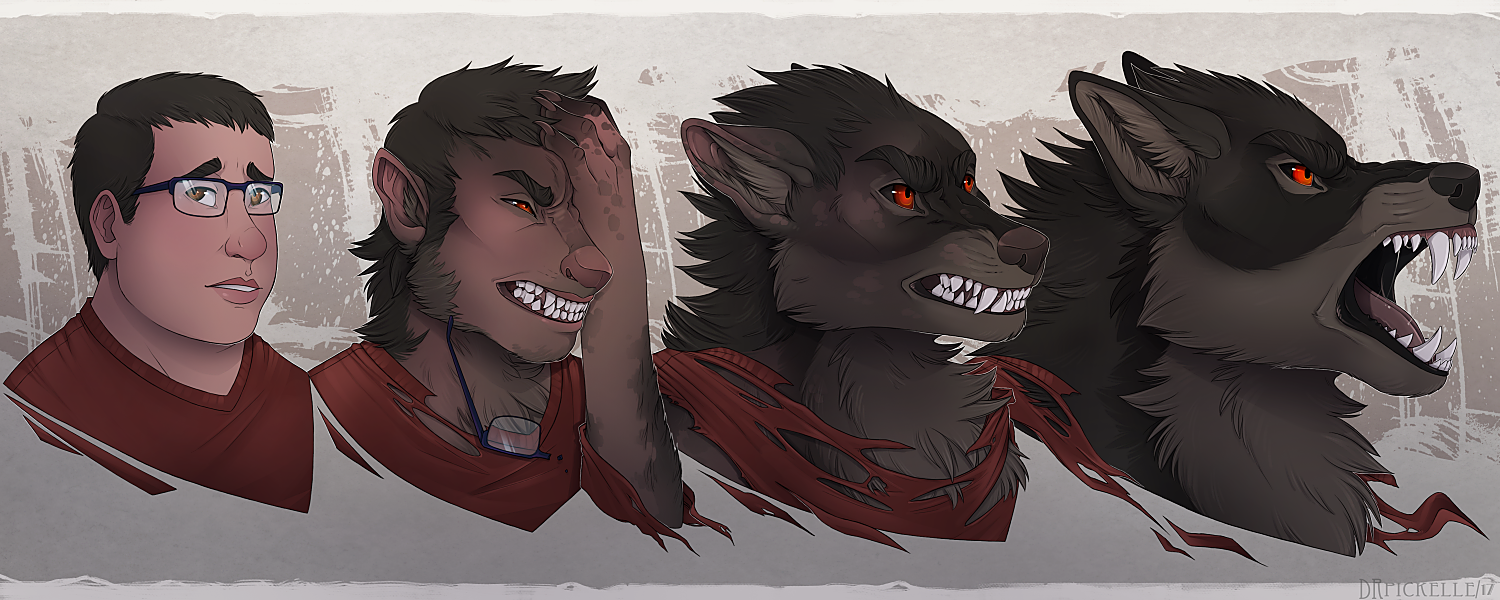The image is a horizontally oriented illustration depicting a four-stage progression of a man transforming into a werewolf from left to right. In the first stage, on the far left, the man is shown from the upper chest up. He is wearing a red shirt, has short dark brown hair, glasses, and a perplexed expression with his eyebrows turned downward. His skin is smooth, and he appears pensive. Moving to the second stage, the transformation begins: his shirt starts to tear, his glasses are broken, longer hair begins to grow, particularly on the sides, and his teeth start to resemble fangs. Additionally, his right hand, now resembling a paw, is raised to his forehead. The third stage reveals a more pronounced werewolf form, with his human features largely replaced by fur. Finally, in the fourth stage, he has fully transformed into a werewolf, characterized by glowing red eyes, an open mouth with prominent fangs, and an overall menacing demeanor as he faces toward the right.